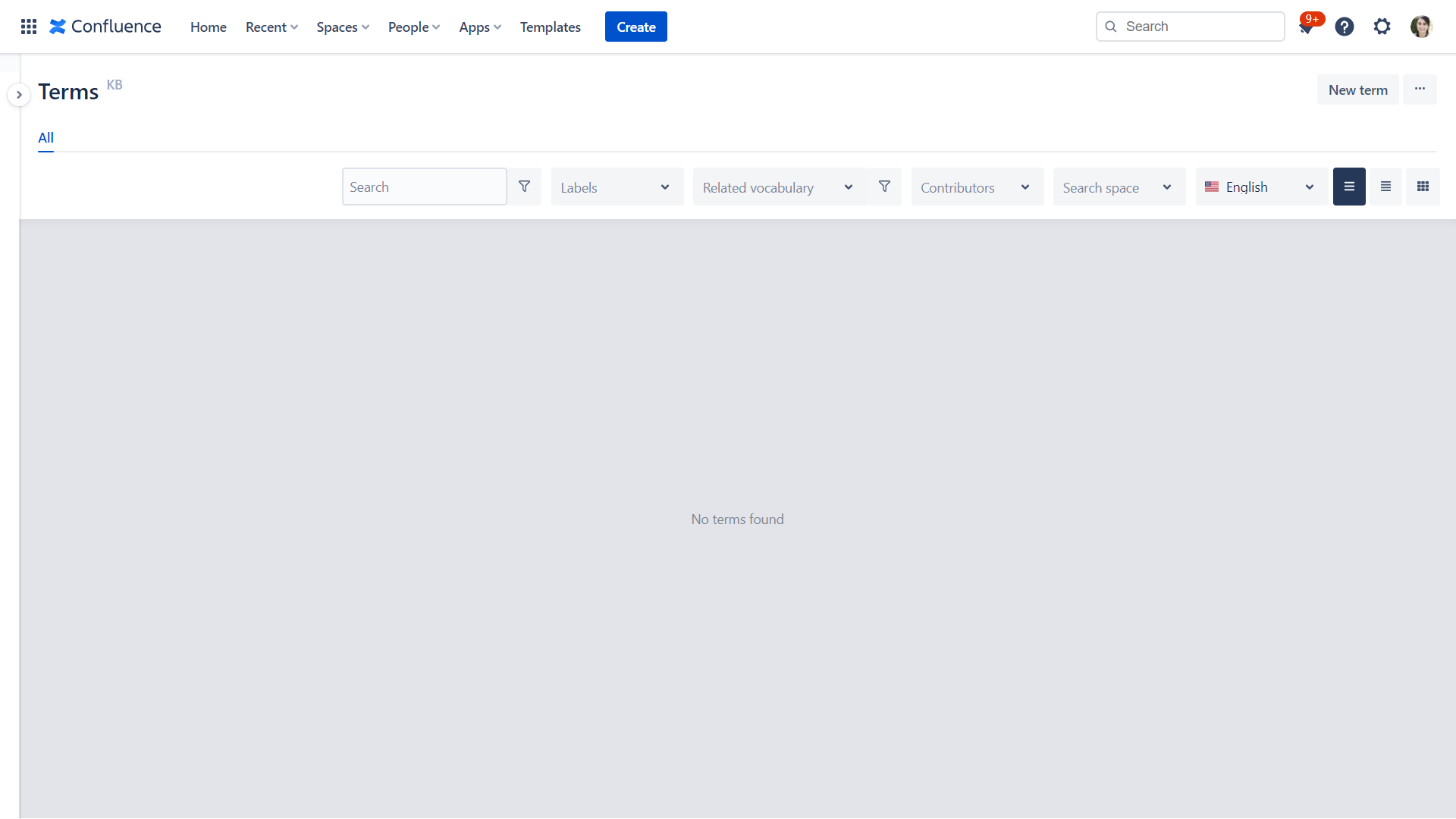The image depicts a detailed interface of an application.

At the top, prominently displayed, is the word "Confidence." Occupying the top-right corner is a navigation banner comprising several options: "Recent," "Spaces," "People," "Apps," "Templates," and "Create." Adjacent to these options is a search bar. Additionally, the user's account is prominently shown with over nine notifications. 

Next to the notifications, icons for "Questions" and "Settings" are visible. Below this navigation area, there is a thumbnail featuring what appears to be a white woman, possibly indicating the account owner.

The subsequent line contains the word "Terms," though its exact purpose is unclear. There is an option to "Create a New Term" and another search bar. Below this are various labels related to the interface: "Vocabulary," "Contributors," "Search Base," and a dropdown menu allowing the user to choose different languages for the interface.

The main area of the screen is primarily grey with a darker grey text in the center stating, "No Terms Found," suggesting that no terms have been searched yet, or the searched term did not yield any results. 

This particular interface appears to be set to the English language.